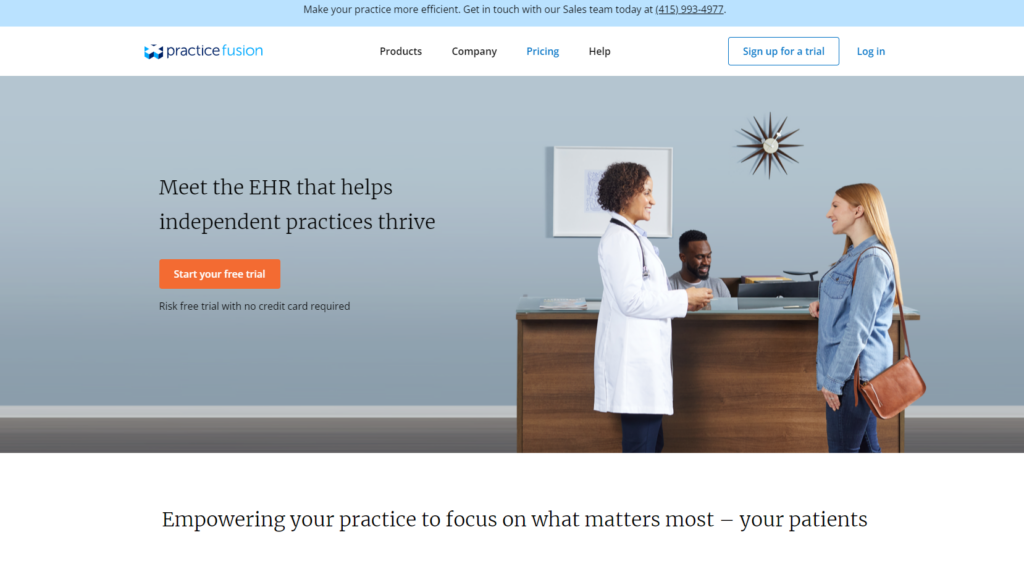In the image, a promotional banner for Practice Fusion's electronic health record (EHR) system is displayed. The top section of the banner features the headline "Meet the EHR that helps independent practices thrive," set against a gray background. To the right, an orange button invites viewers to "Start a risk-free trial with no credit card required." Below this, additional text reads "Empowering your practice to focus on what matters most—your patients."

The backdrop includes elements of a modern medical office, such as a painting on the wall and a clock. A healthcare professional in a white coat with curly hair is shown, exuding a welcoming demeanor. Their attire suggests they are ready to assist in a clinical setting. Adjacent to the promotional materials, various navigation options are displayed, such as "Practice Fusion Products," "Company," "Pricing," and "Health," all set within blue borders.

Overall, the image effectively promotes the EHR system's features and benefits, emphasizing ease of use and priority towards patient care. At the bottom, a call-to-action encourages potential customers to contact the sales team at 415-993-4977 for a more efficient practice experience.